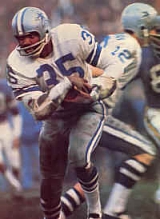The image captures a vintage NFL game featuring the Dallas Cowboys against what appears to be the New York Giants or Minnesota Vikings, though the exact opposing team remains unclear. The central focus is on the Cowboys' player number 35, who is in mid-play after receiving a handoff from player number 12. Player 35, clad in a white jersey with two blue stripes on each arm and the number emblazoned in blue, is preparing to run through the opposing defense. His helmet is silver with a prominent blue star outlined in white, and he wears gray pants with blue and white stripes down the sides, as well as white socks accented with blue stripes. Player 12, also wearing the same uniform, appears to be running in an opposite direction, highlighting the dynamics of the game. The image, likely from the 1970s or early 80s, shows additional players in the background, including one with the number 8 on his jersey. The opposing team members wear dark blue jerseys and white pants, and the scene is set on a gritty, weathered field, adding to the vintage feel of the photograph.